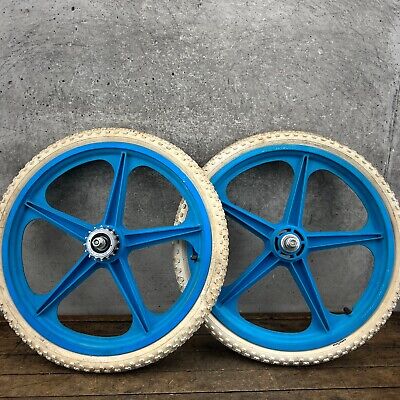The image depicts two bicycle tires leaning against a weathered, gray concrete wall that has a rough texture with white and black splotches, adding to its aged appearance. The tires rest on a wooden floor that resembles old barn wood, with dark, grayish tones. Both tires feature white rubber, and their blue metal spokes form star patterns. The left tire, which shows gears around its center, is positioned slightly in front of the right tire, covering a portion of it. The valve stems of both tires are visible and oriented to the right. The metallic hubs in the middle of each wheel are silver, contrasting with the light blue spokes.